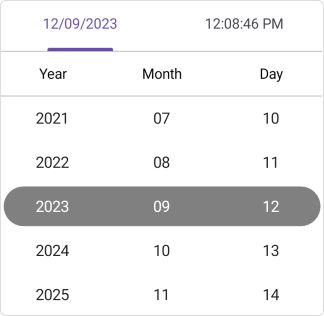The image is a detailed screenshot of a calendar interface taken from a mobile device. The primary focus is on a specific date and time: September 12, 2023, at 12:08:46 PM, displayed prominently in a purple font on the left side. At the top of the calendar, the current year, month, and date are shown in black text, with a scroll option allowing for easy selection of different dates. The selected year is 2023, the month is September (denoted as '9'), and the day is the 12th, all highlighted with a gray bar for clarity. The scrollable options range from years 2021 to 2025, months from July to November, and days from the 10th to the 14th. The calendar has a clean, white background with black font, ensuring all details are easily readable.